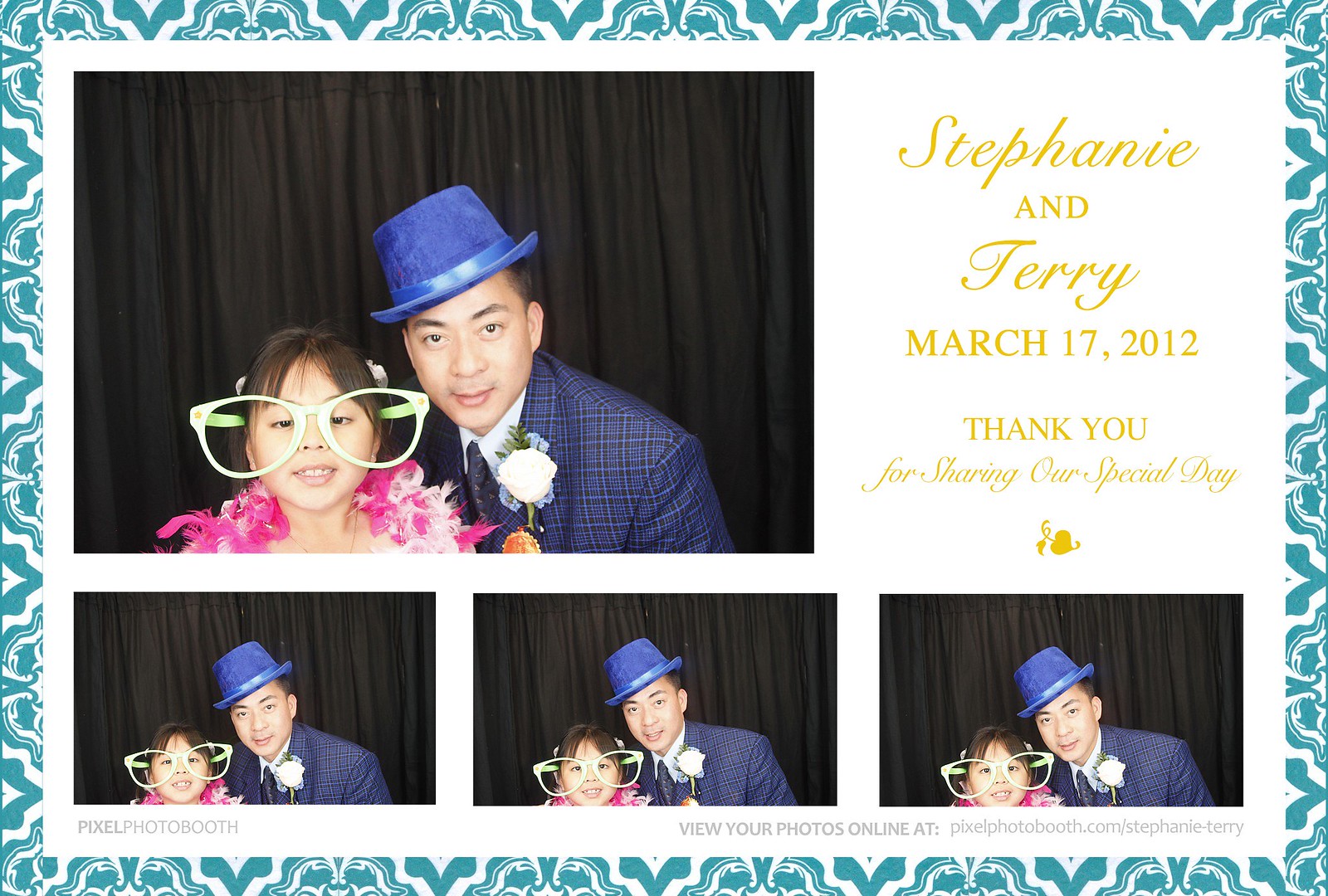The image depicts a decorative poster or invitation card, designed with an elaborate blue and white border. At the center-left, there's a large photograph featuring an Asian man and a young girl, likely father and daughter, participating in a photo booth session. The man is dressed in a blue suit with black checkered patterns, complemented by a matching blue top hat, slightly tilted to the left, and a white flower with a blue outline in his jacket pocket. Standing next to him, the girl wears oversized photography glasses, which appear larger than her head, adding a playful touch to her attire. She also dons a feathered shawl in pink and white around her neck. Below this main image, the identical photo is repeated in three smaller rectangular boxes. The top right corner of the poster displays text that reads, "Stephanie and Terry, March 17, 2012. Thank you for sharing our special day." At the bottom, an additional caption directs viewers to "view your photo online at pixelphotobooth.com/stephanie-terry." The white background accentuates the joyful and celebratory theme, possibly indicating a wedding or similar special event.